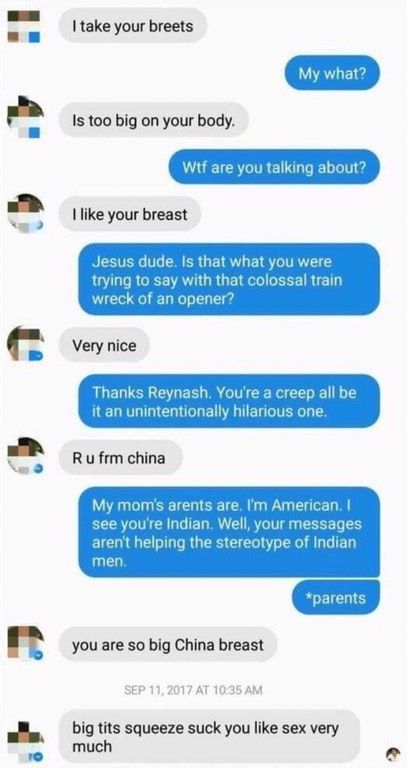**Caption for the Image:**

A detailed screenshot of a text conversation between two people displayed on a smartphone. The image is vertical with a gray border. The messages are organized with each sender's picture on the left, though the pictures are blurred out using small square pixelations. On the right, messages are contained within rounded rectangular boxes, each styled differently depending on who is speaking.

The conversation begins with one person's message in a gray background circular box with the text in black, stating, "I take your breath." The response, in a blue background box with white text, questions, "My what?". The exchange continues with another blue background box asking bluntly, "Is too big on your body." Followed by a response in the same style, "WTF are you talking about?".

Further down, another blue background message inquires, "I like your breast." The answer, in gray with black text, retorts, "Jesus, is that what you were trying to say with that colossal train wreck of an opener?". The conversation continues with awkward and confusing replies. One response reads, "Very nice," another thanks "Ray Nash" with the clarification, "You're a creep, albeit an intentionally hilarious one."

An odd reply in a gray box states, "R U Frm China," followed by a message in a blue box expressing, "My mom's aren't," probably a typo with an asterisk correcting it to "parents."

The chat ends with a time and date stamp from September 11, 2017, at 10:35 AM, and an absurd exchange: "You are so big China breast," followed by a crude statement, "Big kids squeeze suck you like sex very much," highlighting the nonsensical nature of the conversation. There is also a small indistinct picture in the bottom-right corner of the screen.